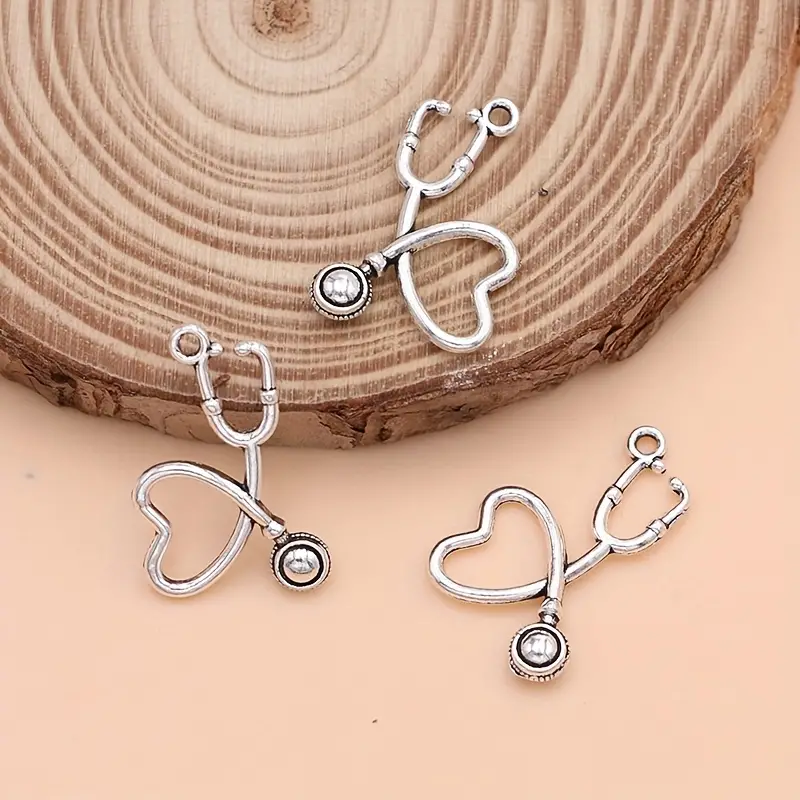The image is a color photograph in a square format, showcasing three identical medical-themed jewelry pieces, possibly earrings or pendants, designed to resemble stethoscopes. The background is a soft peach-pink color. A large, thin wooden slab, cut from the trunk of a tree with visible bark around the edges, occupies the top half of the image. The jewelry pieces are arranged in a visually appealing manner: one lies flat on the wooden slab, another hangs off the edge, draping against the wood, and the third rests on the pink surface. Each charm is crafted from sterling silver and features a stethoscope with the tubing elegantly curved into a heart shape. A silver loop for attachment is located near the earpiece of each charm, and a small clear rhinestone accentuates the chest piece, adding a touch of sparkle. The overall style of the photograph reflects a blend of realism and representationalism, suitable for product photography.